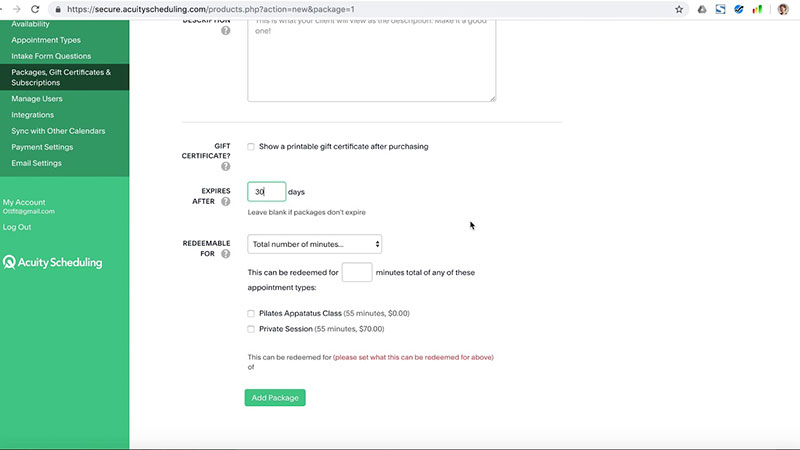This image shows the product description and configuration page for a scheduling website, specifically secure.acuityscheduling.com. At the top, there is a description box where users can input any relevant details they want to display. Below that, there is an option to show a printable gift certificate upon purchase, which is linked to an expiration period currently set to 30 days.

Further down, there is a section labeled "Redeemable For" where users can specify the number of minutes a gift certificate is valid for. This details that the certificate can be redeemed for any selected appointment types. Additionally, two checkboxes are present to select specific types of appointments, such as a 55-minute Pilates or Apetus class, which are listed as private sessions for $0. An option to add a package is also available.

On the left side of the screen, a green column displays various menu options including Availability, Appointment Types, Intake Questions, Packages, Managed Users, Integrations, and more. To the right, there are several icons for additional functions and tools such as a web address field, a star for favorites, a Google Drive icon, a globe icon, a bar graph chart, and a user information icon.